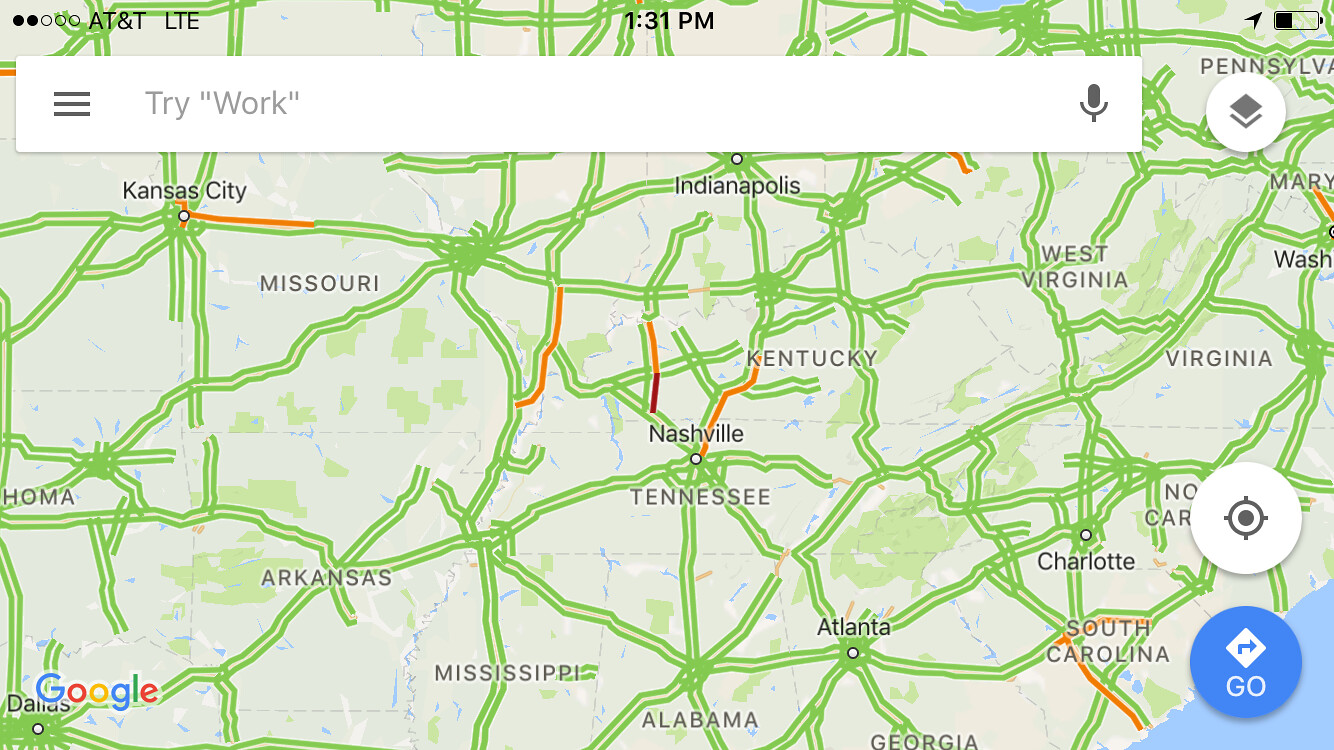The image appears to be a screenshot of Google Maps displaying a detailed map of the southeastern United States. States such as Kentucky, Missouri, Arkansas, Mississippi, Alabama, Georgia, the Carolinas, West Virginia, Virginia, and a portion of Pennsylvania and Washington D.C. are visible. The map contains green lines representing major roads or highways, with several orange lines indicating moderate traffic and a single red line showing heavy traffic.

At the top of the image, there is a white search box with the text "Try work" inside parentheses and a microphone icon at the end, signifying a voice search option. This microphone icon is depicted as a white circle with small dot patterns. The top of the screen also displays the device's status bar, indicating it is 1:31 p.m., the battery level, and that it is connected to AT&T's LTE network.

In the bottom right corner, there is a white circle with a crosshair, likely for location services, and a blue circle with a white arrow symbol labeled "Go," possibly for starting navigation. The bottom left corner features the Google logo, marking the origin of the map service.